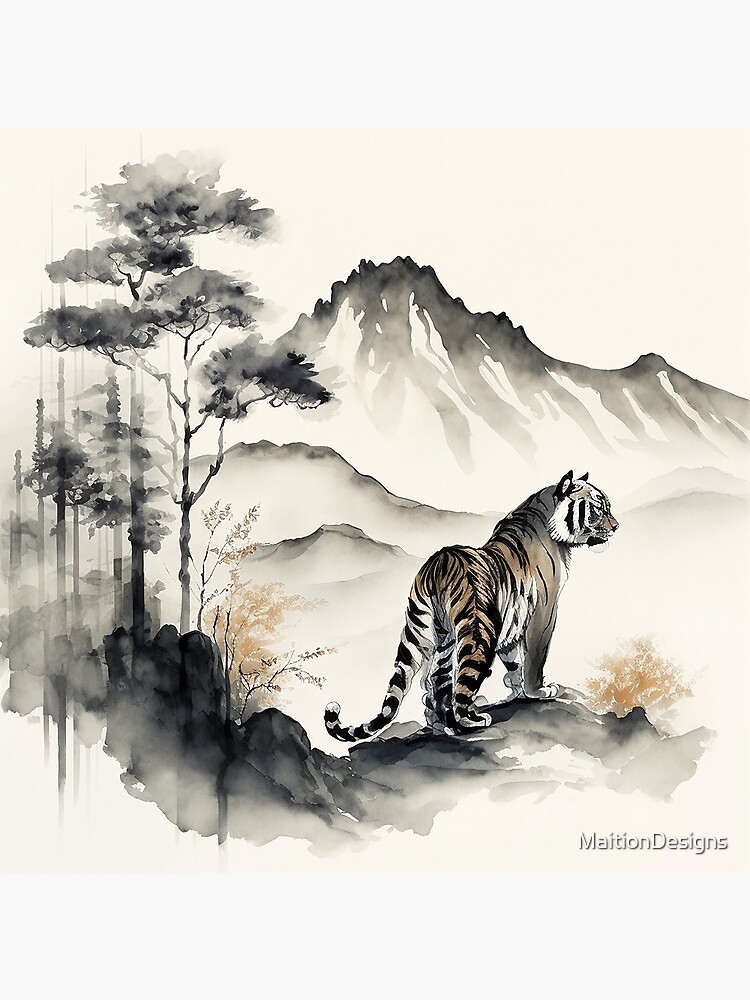This is an exquisite watercolor painting in a traditional Asian style, predominantly rendered in shades of black, white, and gray with subtle hints of brown, tan, and orange. The composition prominently features a majestic tiger standing attentively on an outcropping of rocks in the foreground, its head turned to the right, showcasing its profile with striking black stripes against a brownish-tan coat. The tiger's posture, with its low-hanging tail and intently focused gaze, suggests a moment of poised alertness. To the left of the tiger are wispy trees with sparse leaves, depicted in various shades of gray and black, along with additional rocky formations. Scattered hints of amber and orange in the leaves add a delicate touch of color to the otherwise monochromatic scene. In the background, there is a distant mountain range and foothills meticulously painted in grayscale, creating a sense of depth and vastness in the landscape. The entire scene is set against a white sky, further enhancing the painting's serene and minimalist aesthetic. The painting, hung on an off-white wall, is signed "M-A-I-T-I-O-N Designs" in the bottom right corner, indicating its creation by Maition Designs.